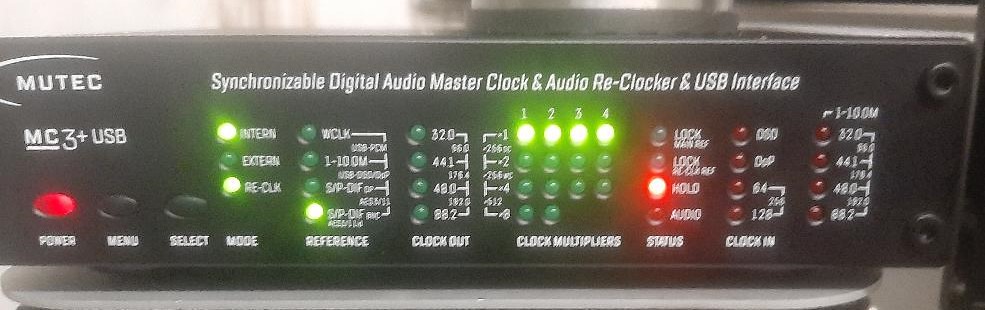The image depicts a rectangular electronic device, branded Mutech (M-U-T-E-C), identified as the MC3+ USB model. Prominently displayed on the front panel, the device is labeled "Synchronizable Digital Audio Master Clock, Audio Reclocker, and USB Interface" in white text. The image shows a variety of illuminated indicators: eight green lights in various columns and rows, with the first four lights at the top lit. Additionally, there is a single red light next to the label "Hold." On the bottom left corner of the device, there are three oval-shaped buttons labeled "Power," "Menu," and "Select," with the Power button glowing red, indicating the device is on. The background of the image is a dark black, emphasizing the detailed and intricate layout of the lights and labels on the device.